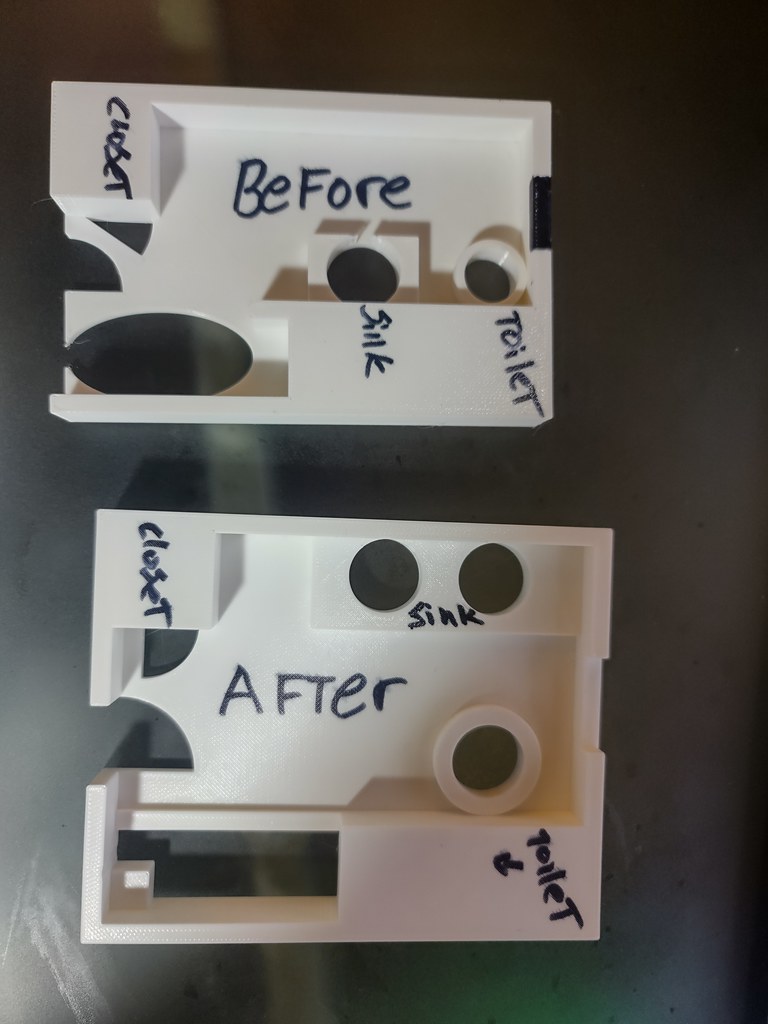In this rectangular image, there is a solid dark-stained wooden desk or countertop serving as the background. Resting on this surface are two notable objects.

The primary object in focus is a rectangular outlet cover displayed from its underside. This cover has various markings created with a black marker to indicate different cutouts and their intended positions. 

Starting from the upper left corner, the word "closet" is written. Moving to the top center, above two small circular cutouts, is the word "before." To the right of these cutouts, the terms "toilet" and "sink" are inscribed. 

Directly beneath this marked outlet cover lies another square cover, also detailed with marker inscriptions. In the upper left corner of this cover, once again, the word "closet" can be seen along with a quarter circle shape adjacent to it. Moving clockwise, there are two circular cutouts now positioned in the upper left area labeled "sink." Near the center, there is a round circle marked "toilet" with an accompanying arrow. Lastly, a rectangular cutout is situated in the lower left of this cover.

This detailed arrangement of the markings on both objects provides a clear indication of their intended placements and functions.